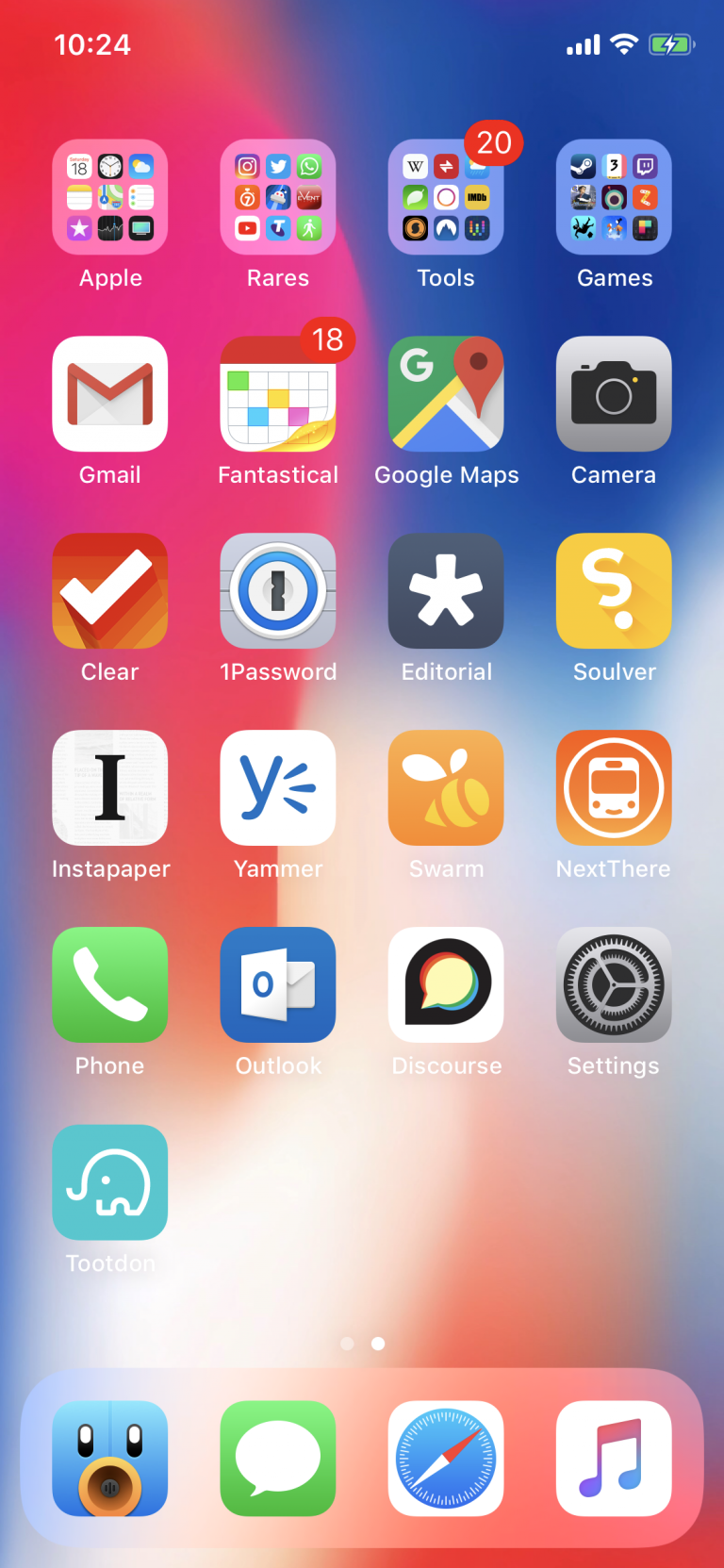A smartphone screen is displayed, showcasing a well-organized and neatly arranged collection of apps. The top left corner of the screen shows the time "10:24," while the top right corner indicates full cellular signal bars, Wi-Fi connectivity, and a green battery icon indicating it is charging. The main screen contains seven rows of apps, each row featuring four apps.

Starting from the top left and moving across the first row, the apps are "Apple," "Rares," "Tools," and "Games." The second row includes "Gmail," "Fantastical," "Google Maps," and "Camera." In the third row, the apps listed are "Clear," "1Password," "Editorial," and "Soulver." The fourth row consists of "Instapaper," "Yammer," "Swarm," and "Next." The fifth row contains "Phone," "Outlook," "Discourse," and "Settings." The sixth row features "TootDon," with only this single app icon, followed by empty space. 

At the bottom of the screen, there are two white dots indicating the presence of multiple home screens, with the current selection on the right dot. 

The dock at the bottom of the screen, which remains constant across all home screens, includes what appear to be four apps. The first icon, which seems to be Twitter, features a blue bird with circular eyes and a beak. Next to it is a green square likely representing WhatsApp, showing a text caption icon. The third icon is Safari, the familiar compass symbol. The description ends without specifying the fourth icon.